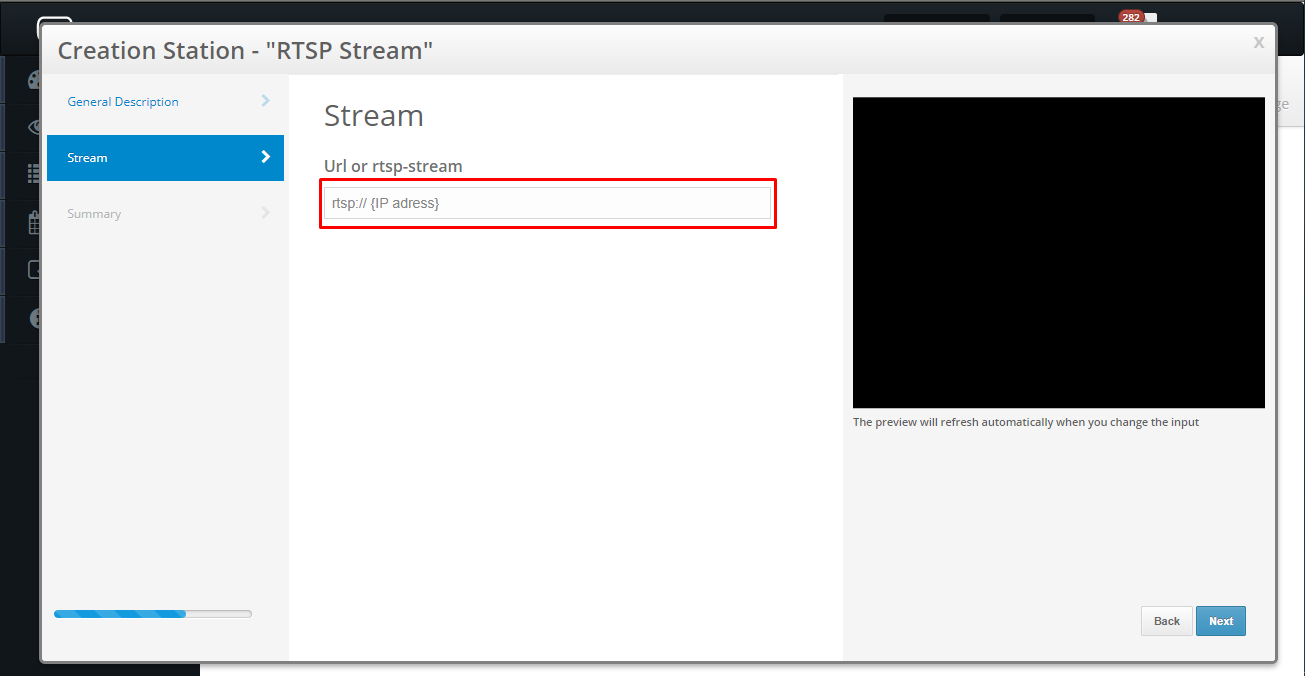This image is a screenshot of a web application, occupying a rectangular and horizontally oriented space on the screen. A black border runs along the far left and across the top edge, while a white border, delineated by a thin vertical black line, defines the right-hand edge. Dominating the center of the screenshot is a large pop-up window with a white and gray background, almost entirely overlaying the primary content.

At the top left corner of this pop-up, the text "Creation Station-RTSP Stream" is prominently displayed. Running vertically down the left side of the pop-up, in blue letters, is the heading "General Description" accompanied by a right-facing arrow. Directly below, the word "Stream," also followed by a right-facing arrow, is highlighted in blue, indicating it is the currently selected section. Below this, the word "Summary" appears in gray font with a right-facing arrow next to it.

Central to the pop-up is the label "Stream," situated above a text box intended for inputting a URL or RTSP-Stream. Adjacent to the right of this box is a black square, possibly a button or an icon. A note at the bottom of the pop-up informs users that "The preview will refresh automatically when you change the input."